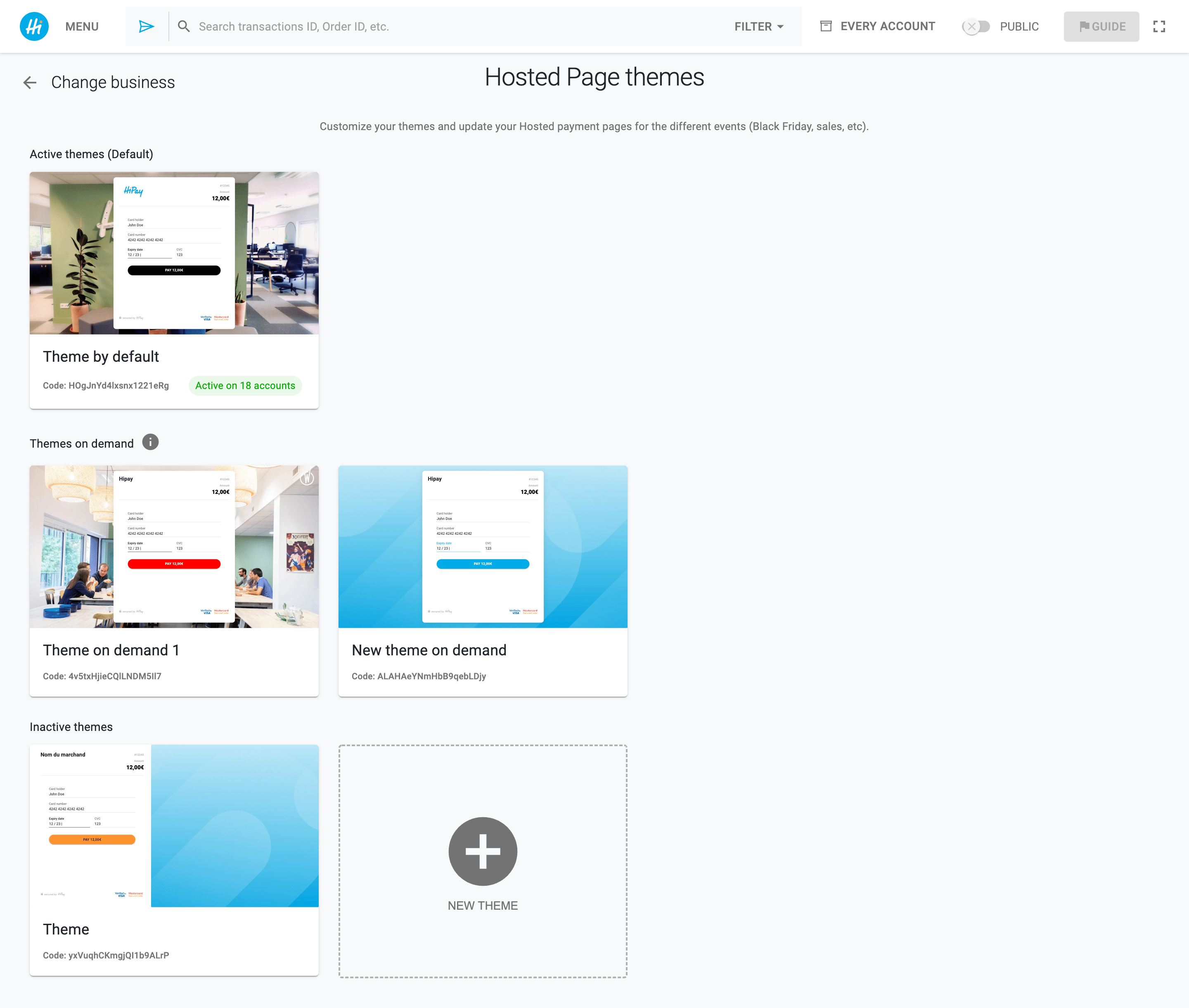This is a webpage showcasing various hosted page themes. The title "Hosted Page Themes" is prominently displayed at the top. The main body of the page features four distinct themes available for selection, each with its unique design and desktop background image. The four themes are: 

1. Default Theme
2. Theme On Demand (Number One)
3. New Theme On Demand
4. Theme

Above each theme description, you can preview the window layout and color scheme associated with that theme. The overall background of the webpage is white, creating a clean and minimalistic appearance.

In the top left corner, there is a menu button next to the company's logo, which consists of a blue circle with white lettering inside. To the top right, there are several interactive buttons, including a filter button, an account view button, and a toggle button to switch between public and private views. The right side of the page features a large, empty white space.